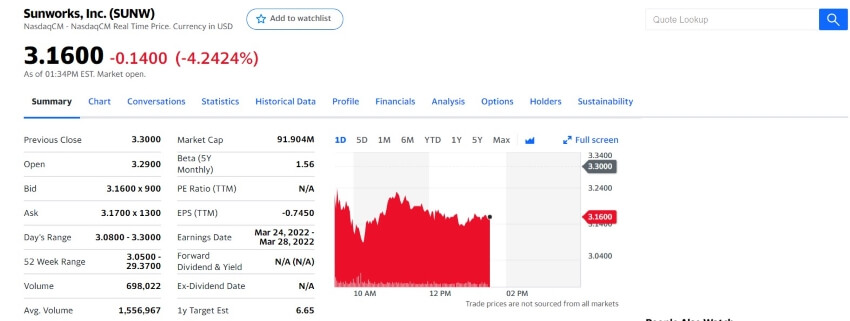Screenshot Description: Detailed Stock Update for Sunworks Inc. (SUNW)

The image is a detailed screenshot of a stock update interface, specifically for Sunworks Inc., a company identified by the stock ticker symbol SUNW. 

Starting from the top left, the company name Sunworks Inc. is prominently displayed, with its ticker symbol (SUNW) shown in parentheses immediately after. Directly below the company name and symbol, the current stock price is listed as 3.1600. Positioned to the right of this price, in red text, is a negative change of -0.1400, indicating a decrease in the stock value. Further illustrating the decline, a percentage change of -4.2424% is also displayed in red within parentheses.

Below the stock information, various navigational categories are listed, aiding in detailed analysis and data retrieval. These categories include:
- Summary
- Chart
- Conversations
- Statistics
- Historical Data
- Profile
- Financials
- Analysis
- Options
- Holders
- Sustainability

On the left side of the screenshot, different stock metrics are organized under specific sections for comprehensive insights, including:
- Previous Close
- Open
- Bid
- Ask
- Volume
- Market Cap
- Beta
- P/E Ratio
- EPS
- Earnings Date

Each section provides a concise yet thorough overview of Sunworks Inc.'s current stock status, facilitating a complete analysis for investors or analysts monitoring SUNW.